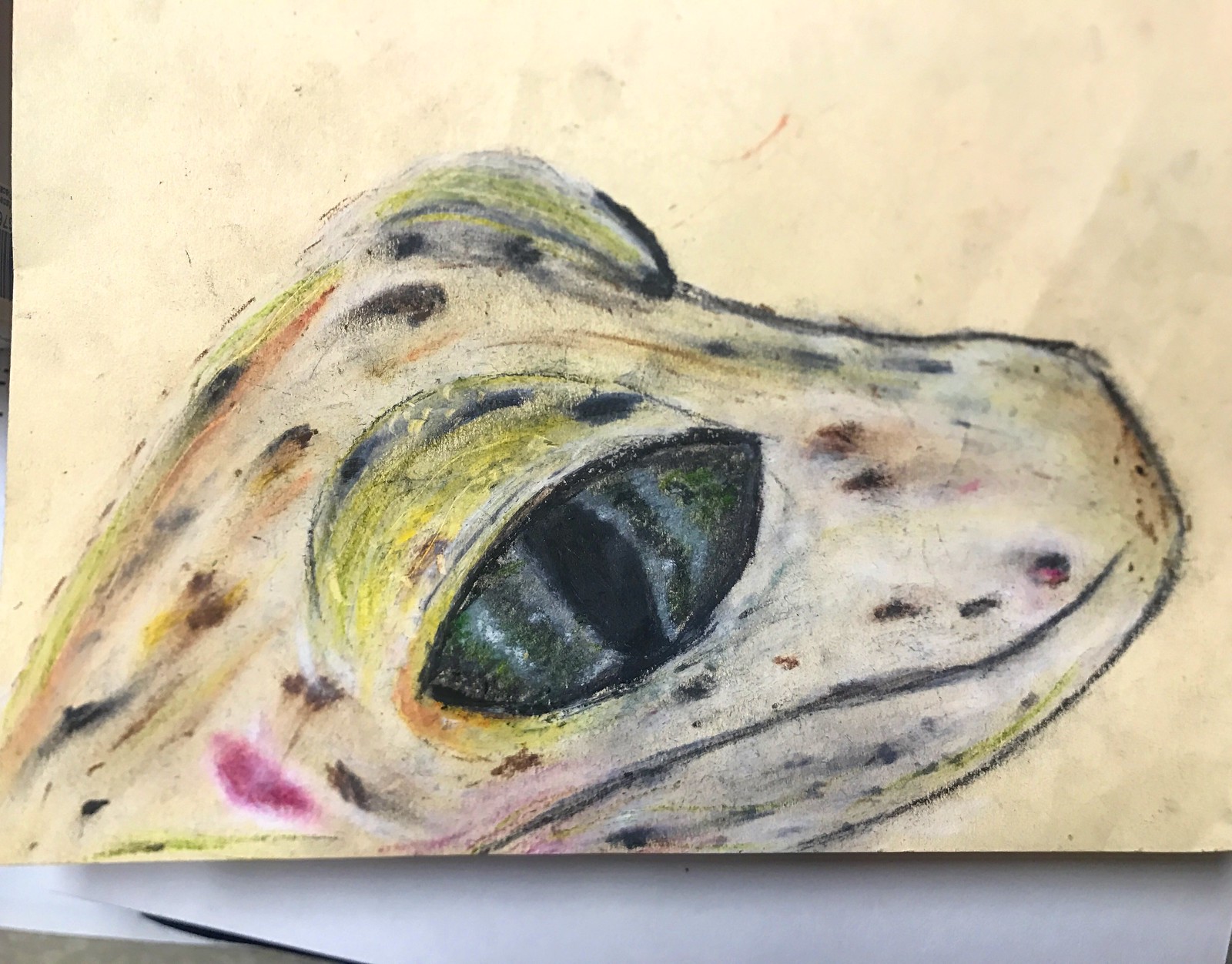This artwork vividly captures the head of a lizard, meticulously illustrated using either colored pencils or watercolors. The lizard, rendered in delicate hues of light beige and yellow, is adorned with subtle black spots that enhance its lifelike appearance. Emerging from the bottom left corner of the page, the lizard's head is elegantly positioned upward and facing right. A striking feature is its prominent, wide eye, reminiscent of a cat's eye, with a rounded top that adds an intense, observant gaze. The background complements the subject with a soft, light cream color, seamlessly highlighting the intricate details of the lizard. This piece beautifully showcases the artist's skill in bringing the reptile to life with both texture and depth in a serene, natural setting.